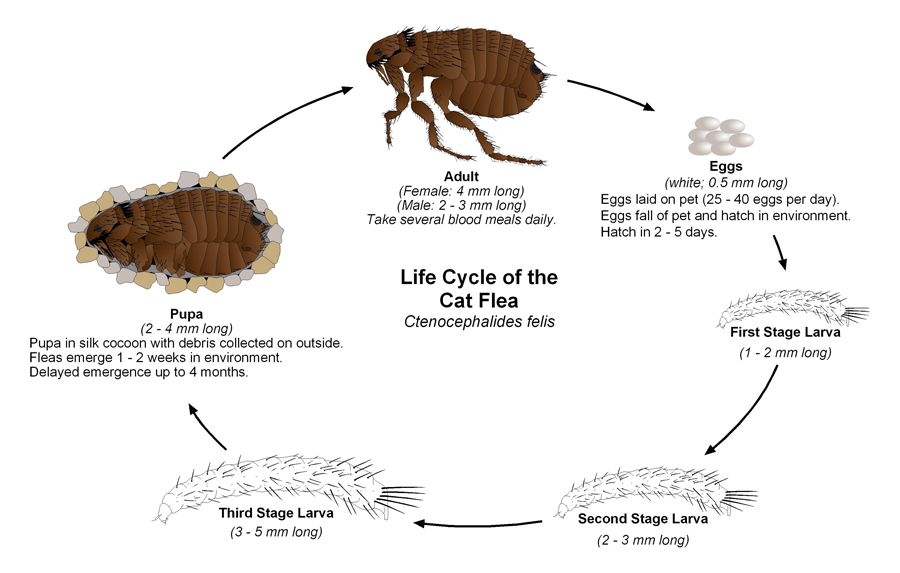The image is a detailed diagram illustrating the life cycle of the cat flea, featuring the title "Life Cycle of the Cat Flea" along with its Latin name, on an immaculate white background without visible edges. It presents a clockwise sequence of the six life stages in black text accompanied by descriptive images. At the top, the cycle begins (or ends) with the adult stage, depicting a brown flea labeled as "Adult," providing details about its length (4 mm for females and 2-3 mm for males) and dietary habits (several blood meals daily). An arrow leads to the "Eggs" stage, capturing approximately six to seven eggs grouped together, noting that fleas lay 25 to 40 eggs daily on the host, which fall off and hatch in 2 to 5 days. Next is the "First Stage Larva," shown as a small, oval creature with hairs, followed by the "Second Stage Larva," slightly larger with more details. The transition continues to the "Third Stage Larva," the largest of the larval stages with even more pronounced hairs. The subsequent stage is the "Pupa," illustrated in a silk cocoon collecting debris, indicating emergence in 1 to 2 weeks, with a potential delay up to 4 months due to environmental factors. The cycle completes as an arrow directs back to the beginning stage of the adult flea. The predominant colors in the diagram are black and white for the initial stages and brown for the pupa and adult flea, enhancing visual comprehension of each phase.